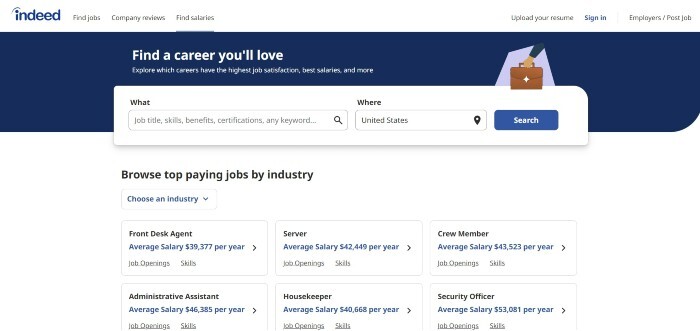The image captures a screenshot of the Indeed website, prominently displaying the Indeed logo in the top left corner set against a navy blue navigation bar. In this navigation bar, users can make use of a search function that allows them to specify job criteria. The search fields provided include "what" where you can enter a job title, skill, certification, benefit, etc., and "where" to define a location such as "United States." A blue search button with the text "Search" in white is present to execute the search.

Below the search bar, an additional feature offers users the ability to browse top-paying jobs by industry. A drop-down menu facilitates the selection of an industry, subsequently displaying typical salary levels, current job openings, and the skills required for those positions. Six listed examples of job titles are shown: Front Desk Agent, Server, Crew Member, Administration Assistant, Housekeeper, and Security Officer. From this list, the role of Security Officer stands out with the highest average salary, exceeding £53,081 per year.